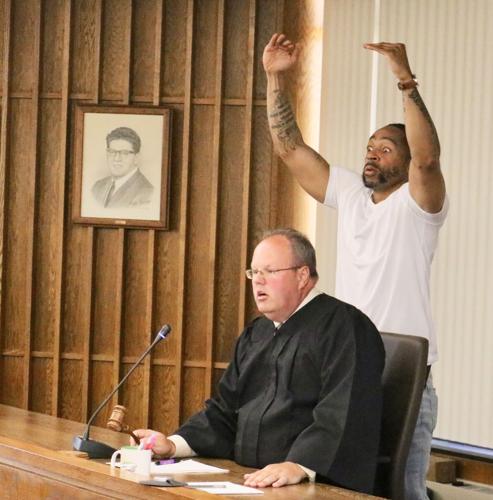The image is a color photograph depicting a courtroom scene. At the center of the photograph is a judge sitting on the bench. The judge, an older white man with thinning hair and glasses, is wearing a black robe and sitting in a black chair. In his hand, he holds a gavel, while his other hand rests on a large wooden desk that holds a pad, pen, coffee mug, and a microphone. Behind the judge, a bald man stands with his muscular, tattooed arms raised over his head. This man is dressed in a short-sleeved white t-shirt and blue jeans, with a beard and mustache, and he has a look of surprise on his face as he gestures towards the courtroom. The background of the scene includes a wall with wood paneling adorned with a monochrome portrait of a man in glasses and a suit. To the right, there is a window covered with white blinds. The setting emphasizes a formal courtroom environment, capturing the tension and drama of the moment.